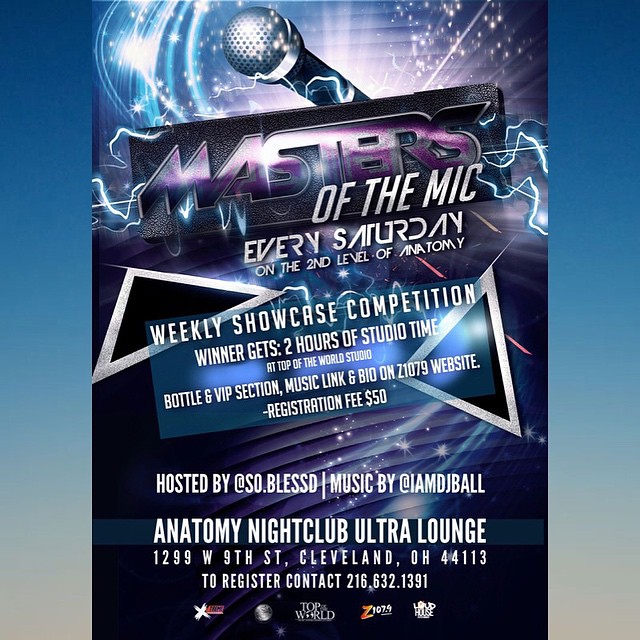This image is a detailed advertisement for an event at a nightclub and lounge, specifically the Anatomy Nightclub Ultra Lounge located at 1299 West 9th Street, Cleveland, Ohio, 44113. Dominating the top of the image is an electrified microphone with lightning striking through it, evoking a high-energy vibe with starry and cloud-like metallic colors in the background. 

Centrally, in bold purple letters against a black background, the title "MASTERS" stands out, followed by "OF THE MIC" beneath it. Below, information about the event is clearly displayed: "Every Saturday on the second level of ANATOMY," and "WEEKLY SHOWCASE COMPETITION" in white letters against a blue backdrop. 

Important details include prizes for the competition winner, such as 2 hours of studio time at Top of the World Studio, a bottle, access to a VIP section, and a music link and bio feature on the Z107.9 website. There's a registration fee of $50, and the event is hosted by SoBlessed with music by DJ IamDJPaul. 

Contact information for registration is provided at the bottom, listing the number 216-632-1391. The logos for Top of the World Studio and radio station Z107.9 add authenticity and further details to the image. All these elements combined create a vivid and thorough description of a captivating night of competitive entertainment.